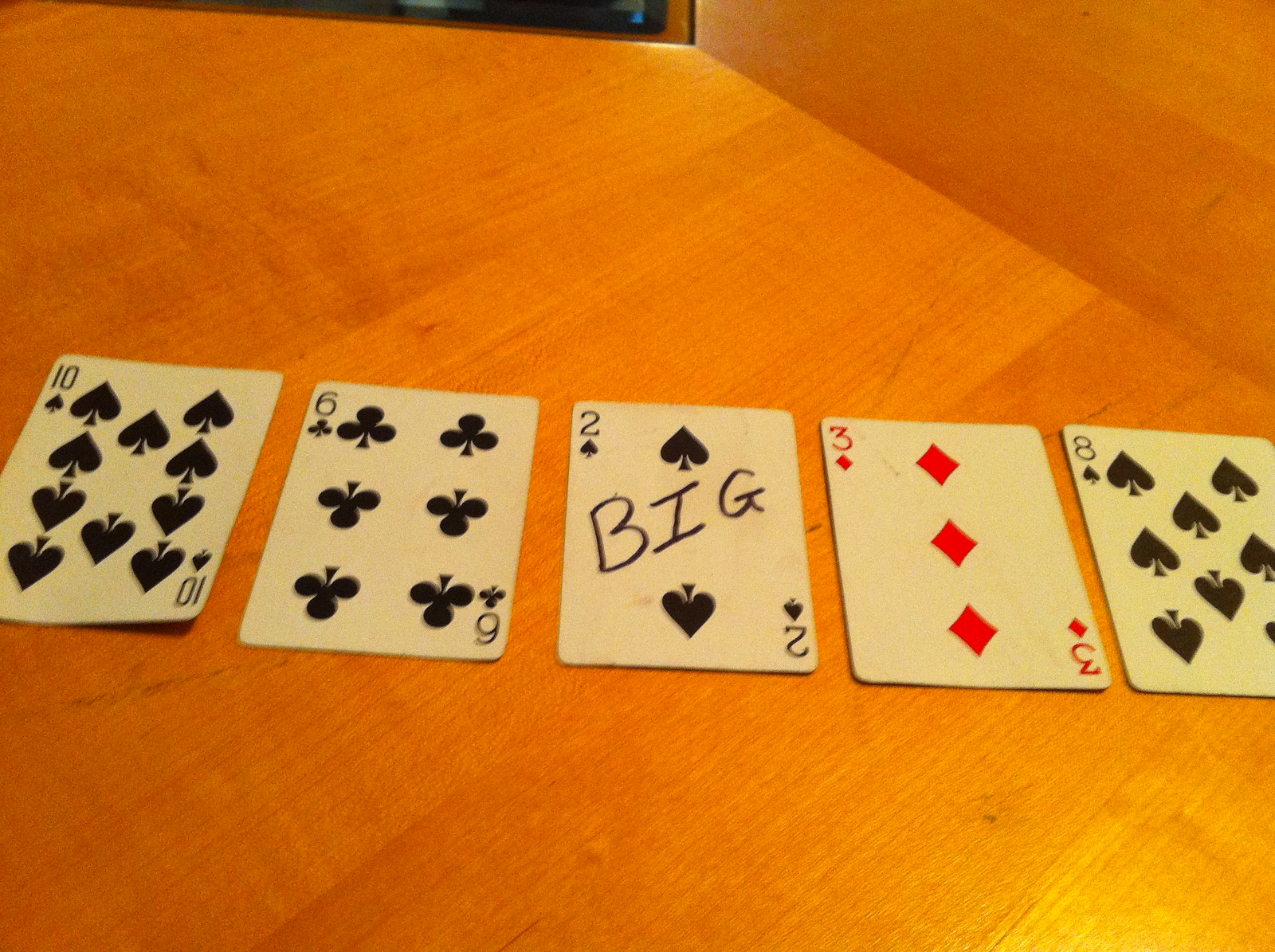This color photograph features a detailed arrangement of five playing cards, neatly laid out side-by-side to form a horizontal row. The cards rest on a medium brown wooden surface, infused with subtle golden undertones. In the upper right corner of the image, we see the edge of what appears to be a bookshelf or possibly a side wall. 

The playing cards, listed from left to right, are the Ten of Spades, the Six of Clubs, the Two of Spades, the Three of Diamonds, and the Eight of Spades. Notably, the Two of Spades is marked with the word "BIG" written diagonally across the card in capital letters, using what seems to be a black magic marker. 

A thin sliver of the background is visible at the very top of the photograph, showing a turquoise blue strip of color, with the rest of the background fading into black.